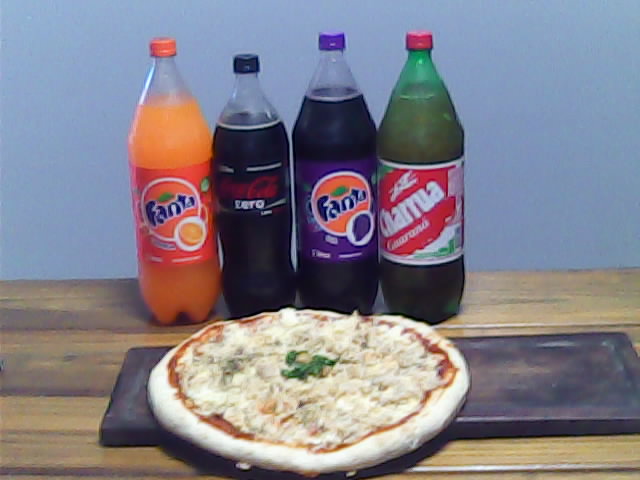The photograph depicts a small rectangular black tray centered on a wooden brown table with visible boards, set against a light blue background. On the tray, there is an uncooked cheese pizza with a white crust and un-melted white cheese, sprinkled with basil in the middle. The pizza, which overhangs the tray slightly, appears somewhat blurry. Positioned behind the pizza are four large soda bottles arranged from left to right: an Orange Fanta, a Coca-Cola Zero with a black label, a Grape Fanta with a purple label and an orange logo, and a Charrua Guaraná in a green bottle with a red cap and red logo.